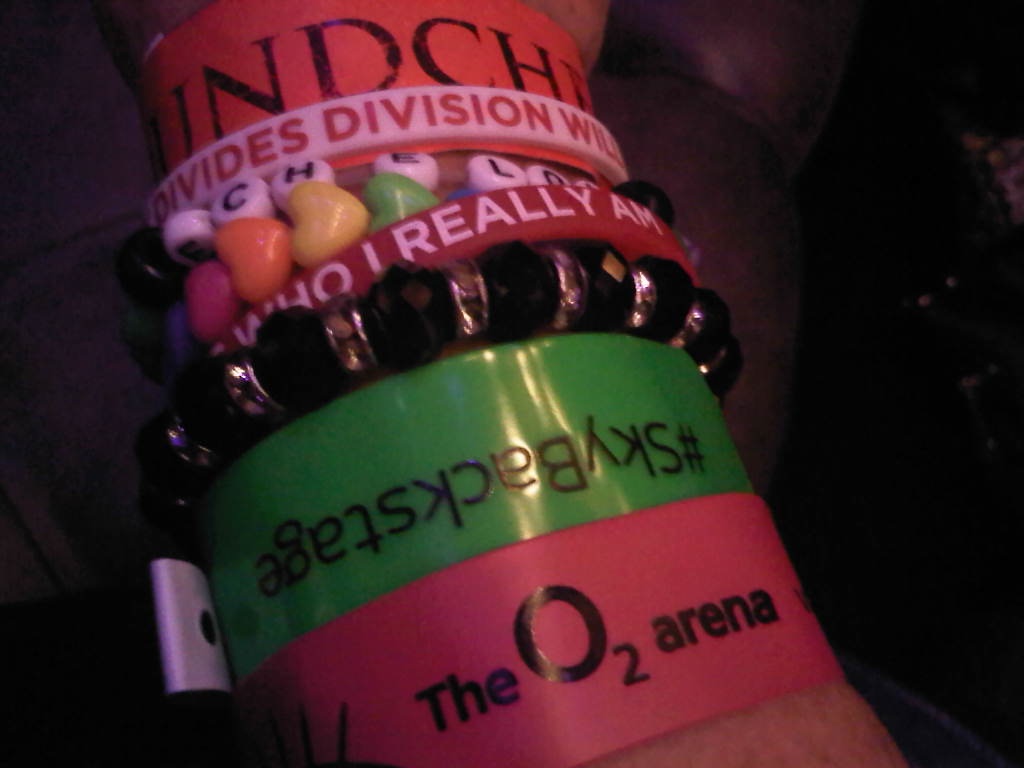This low-quality, slightly grainy color photograph captures a close-up of a person's wrist adorned with a variety of colorful bracelets, each bearing different text and designs. Starting from the top, the wrist features an orange plastic bracelet with the text "I-N-D-C-H." Below it, a white thinner band reads "divides division will" in red lettering. Descending further, there is a bracelet made of letters followed by a plastic bracelet with a rainbow heart design. Next, a thin red bracelet displays the partially visible text "who I really am." Lower on the wrist lies a rhinestone bracelet composed of black and silver beads, adding a touch of shine. Toward the bottom of the image and extending closer to the elbow, the wrist holds two thicker plastic bracelets: a green one inscribed with "#sky backstage" and a pink one that reads "the O2 arena." The wrist and bracelets appear slightly blurry against a dark, indistinct background, rendering further details indistinguishable.